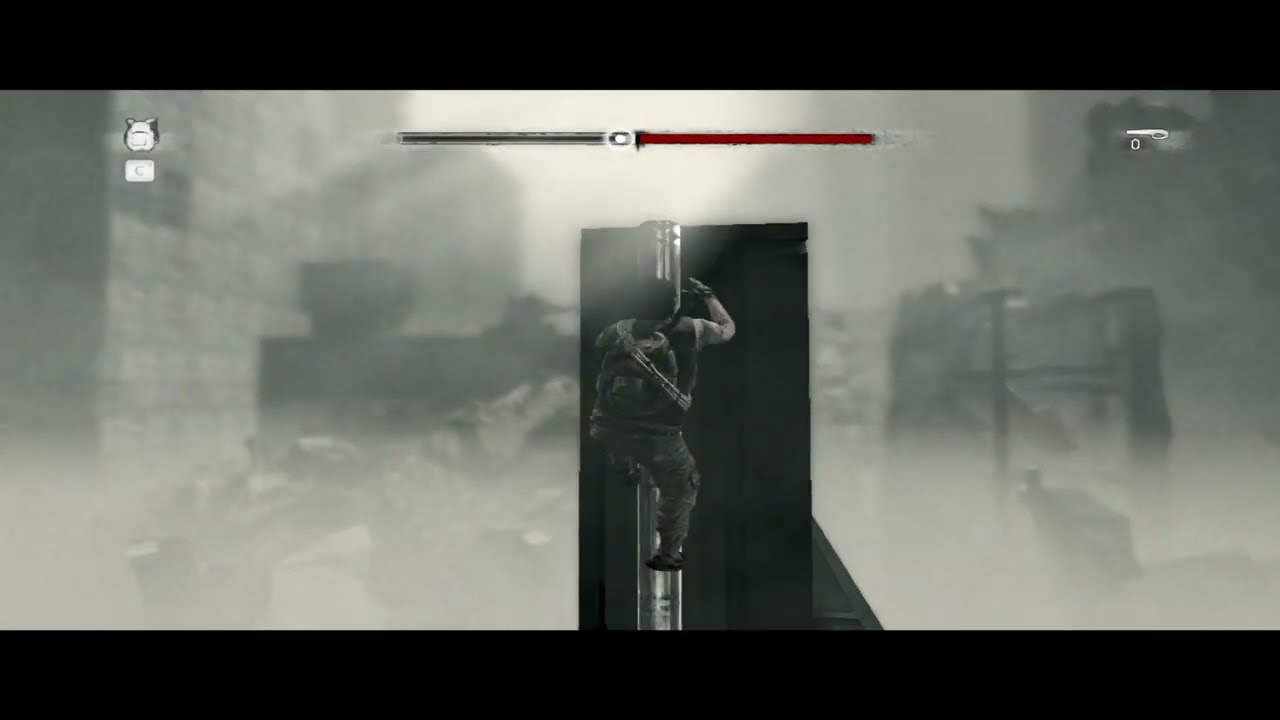The black and white digital image, horizontally rectangular, features a thick border on the top and bottom but not on the sides. The background is gray and out of focus, resembling rubble or broken-down buildings, contributing to a smoky and indistinct appearance. At the center of the image, a man dressed in fatigues and a short-sleeved shirt is climbing a structure, possibly a pipe or ladder, on the side of a building. He carries a heavy-duty backpack and wears gloves. Above him, a progress bar spans the top of the image, with one half black and the other half red, featuring a marking in the center—a white area with a black "C" symbol. The overall scene is reminiscent of a video game screen, with diffused lighting suggesting a white sky section. The left side of the image indicates a stone wall, while various indistinguishable items populate the lower portion amidst the blurry background.